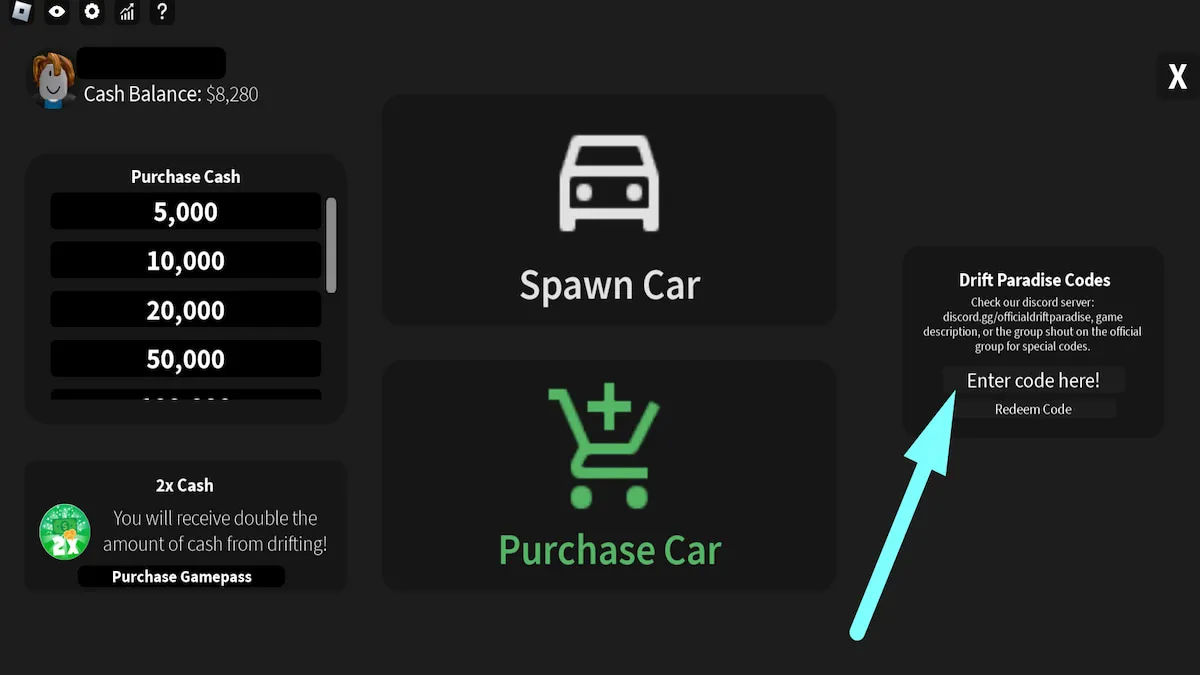The image displays a user interface with a black background, featuring a menu and various controls related to an application that seems to involve stocks or cars. 

**Top Left Corner:**
- A series of options are visible, likely related to user interactions with stocks or cars, though the specifics are unclear.

**Description Panel (Left side):**
- There is an emoji of a brown-haired, white, smiley-faced individual adjacent to the text "Cash Balance: $8,280."
- Below the cash balance, there's a "Purchase Cash" section offering different amounts of cash, listed as $5,000, $10,000, $20,000, $50,000, etc.
- At the bottom left, a button labeled "2X Cash" notes, "You'll receive double the amount of cash from drifting," with an option to purchase a game pass.

**Central Section:**
- Two black boxes dominate the central area:
  - The top box features an image of a white car with a label "Spawn Car."
  - Adjacent is a green shopping basket icon with a plus sign, labeled "Purchase Car."
  
**Directional Arrow:**
- Extending from the bottom center to the top right, a light blue arrow points to another black box.

**Right-Hand Box:**
- This black box is titled "Drift Paradise Codes."
- It instructs users to check the Discord server for special codes, providing a website link.
- The description suggests checking the game description or group shout on the official group for codes, with a field to enter and redeem a code.

**Upper Right Corner:**
- A white "X" icon is present, likely to close the settings or interface window.

Overall, the interface aids in navigation, cash management, car spawning, and entering promotional codes for the game or application being described.